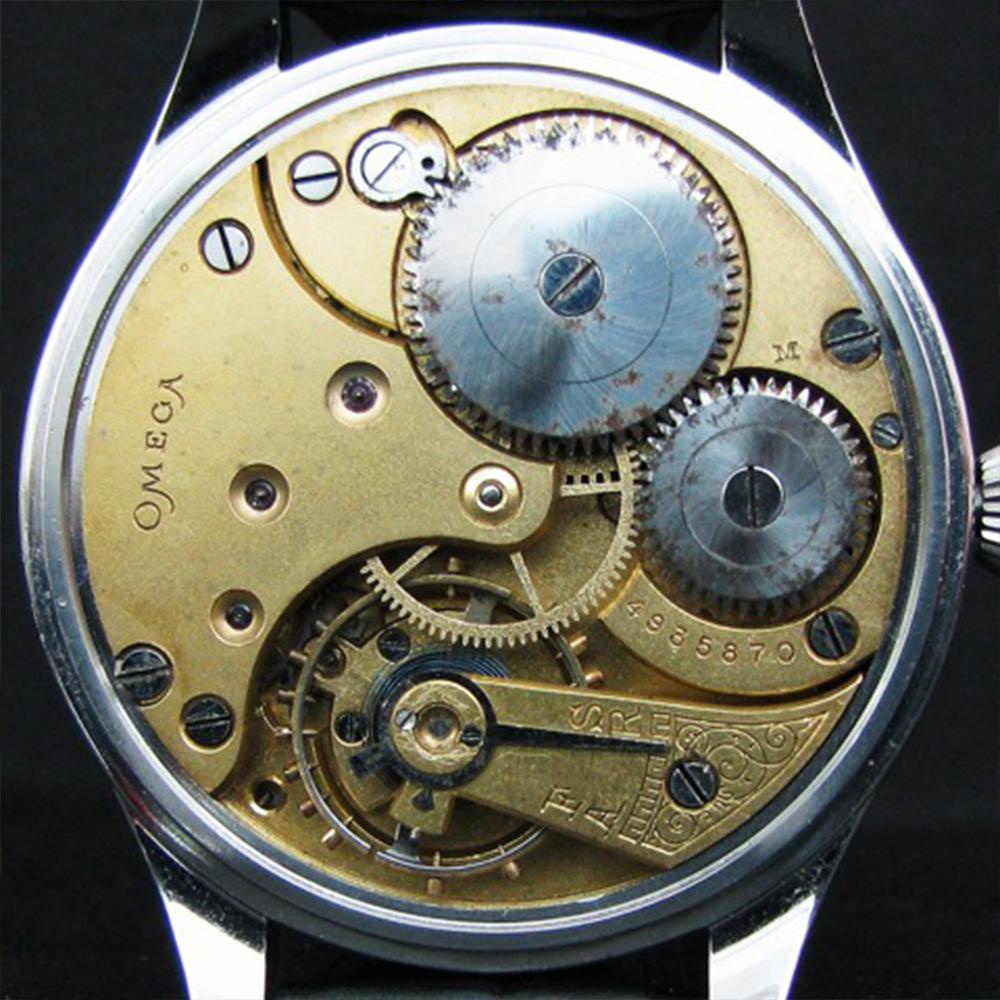This image highlights the intricate mechanisms of a high-end Omega wristwatch against a stark black background. Dominating the square frame, the watch's back cover has been meticulously removed, revealing a circular interior with a shiny silver perimeter. The inner workings are a striking contrast of gold and silver components. The gold base showcases various gears, some appearing rusty from probable past exposure to moisture. Notably, the upper half features a prominent large gear, accompanied by smaller silver gears to its right, near the dial. Protective gold plates guard additional gears, maintaining the watch's sophisticated aura. The brand name "Omega" is inscribed vertically on the left, signaling its premium quality. The delicate interplay of silver screws and gears, some gold, reflects both precision craftsmanship and the passage of time.